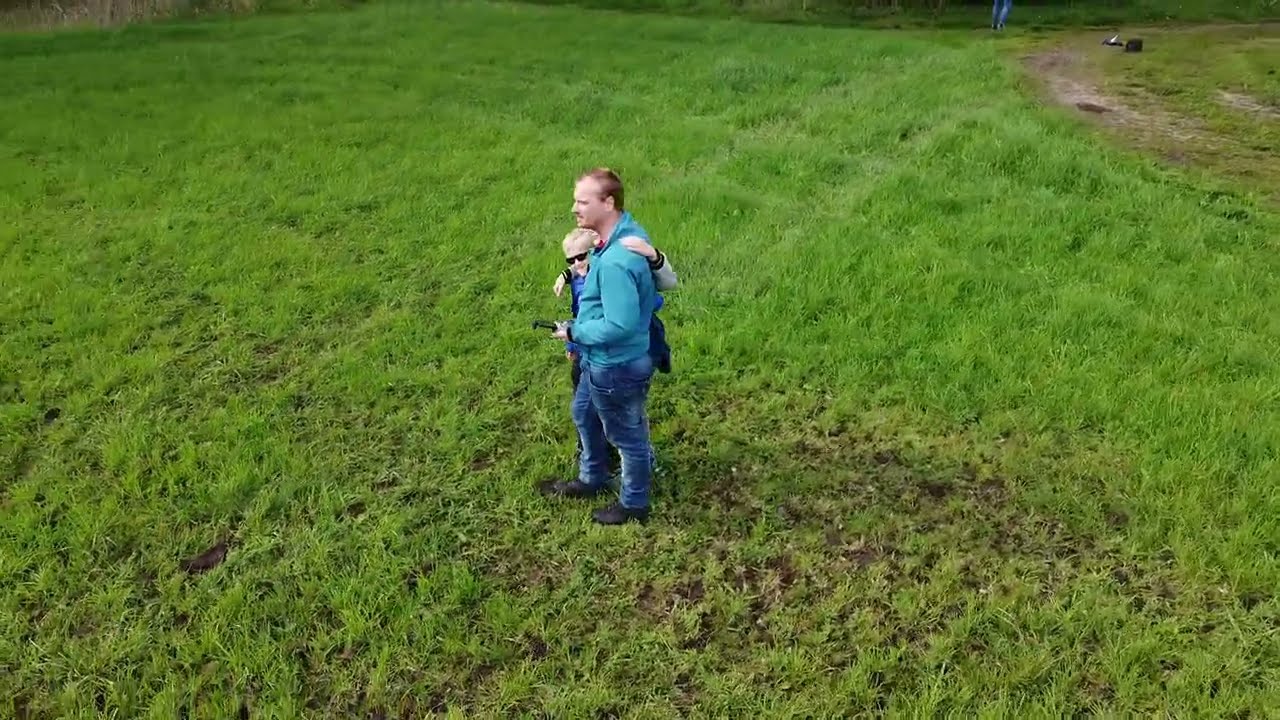In this photograph, a middle-aged man, possibly in his late 30s or early 40s, stands prominently in the center of a lush, green grassy field. He is wearing a blue long-sleeve shirt, navy blue jeans, and black cowboy boots. His receding brownish-red hairline almost reaches his ears. The man faces left, gazing off towards the edge of the photo frame with an enigmatic expression.

On his right side, partially concealed by the man's body, is a young child who appears to be his son. The child, adorned with black sunglasses and sporting blonde hair, joyfully drapes his left arm over the man's left shoulder, offering a warm, affectionate hug that warms the scene. The child's head peeks out, looking directly at the camera with a cheerful demeanor, while his body remains mostly hidden behind the man.

This touching family moment is captured from a slightly elevated angle, allowing the viewer to take in the expanse of the verdant field around them. Though the primary focus is on the man and his son, a subtle detail—a pair of legs—can be seen at the top right corner of the image, adding a hint of mystery to the serene landscape.